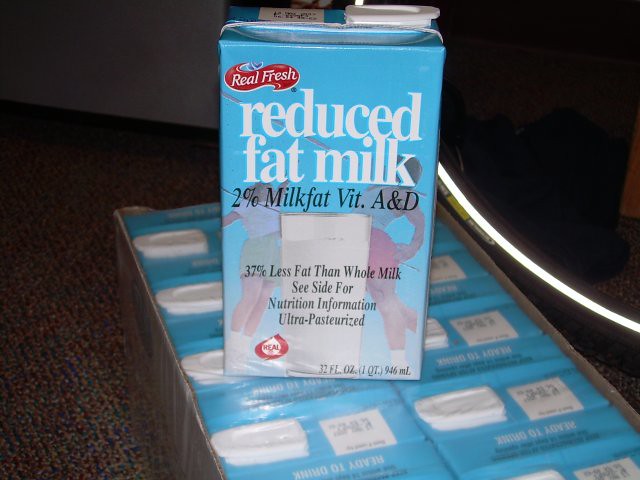This photograph features a close-up of a small, single-serving box of Realfresh brand reduced-fat milk. The box is predominantly light blue, with large white letters displaying "Reduced Fat Milk" prominently on the front. Below this, in black text, it states "2% milk fat, Vitamins A and D." Further down, the text indicates "37% less fat than whole milk," and advises to "See side for nutritional information." The milk is ultra-pasteurized, and there's a red-and-white "Real Milk" logo in the bottom left corner, along with a "Real Fresh" logo at the top. The box also features an image of a minotaur and a glass of milk. The small milk box is situated on a case that contains several other identical boxes, wrapped in plastic like a carton. To the right of the image, part of a bike tire is visible, while to the left, there's a tan carpet with blue woven in, and a white wall in the upper left corner.